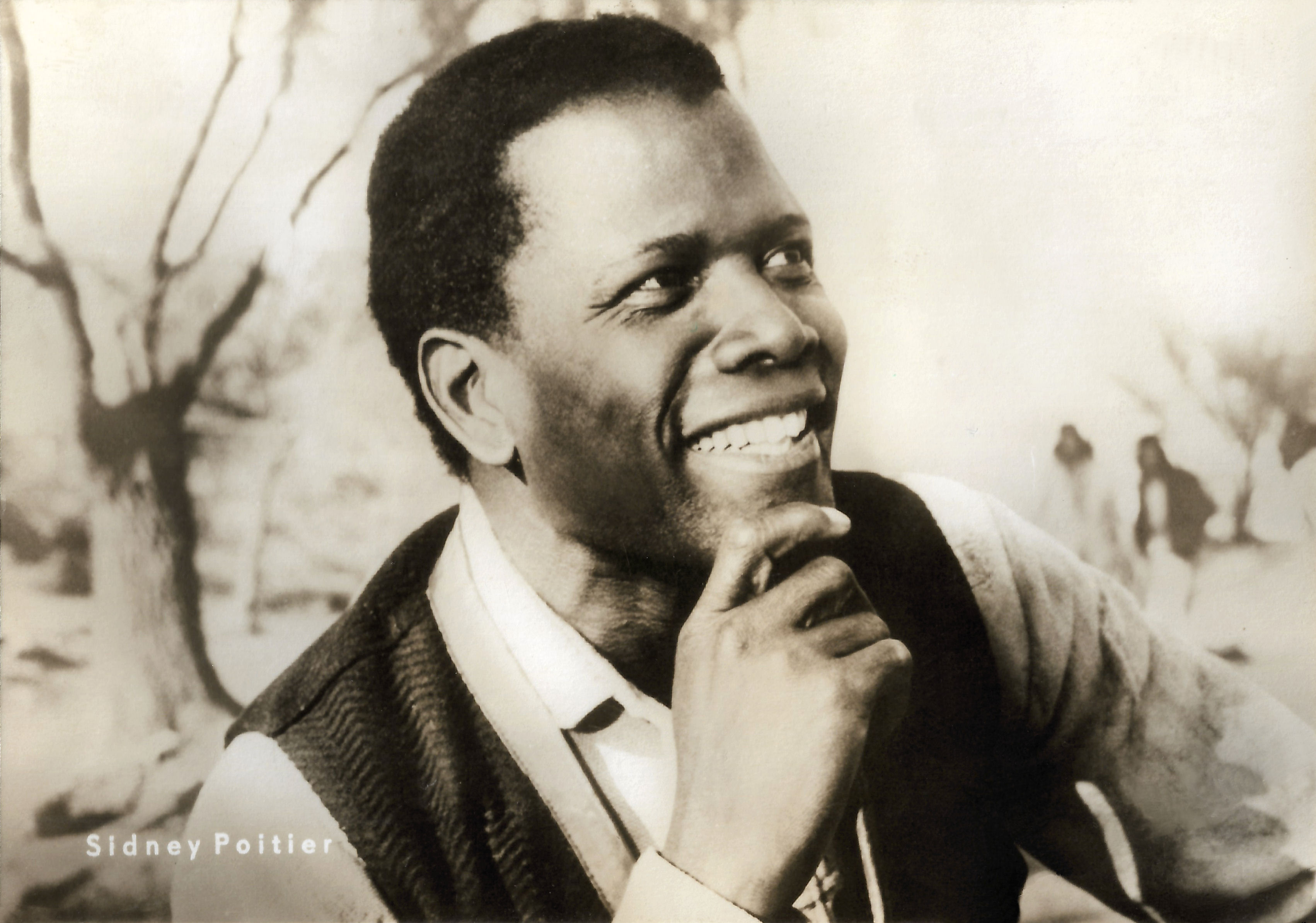In this black and white photograph, Sidney Poitier is captured looking towards the upper right corner with a contemplative expression. His body is slightly angled to the right, and his right hand is thoughtfully placed near his chin. Poitier, radiating a warm smile that highlights crinkles around his mouth and eyes, showcases both his top and lower teeth. His short, curly black hair complements his stylish outfit: a textured black vest over a long-sleeve coat, beneath which he wears a light-colored, button-up shirt with the top two buttons undone. His left arm extends slightly forward. In the bottom left corner of the image, the name "Sidney Poitier" is prominently displayed in white text. The background reveals a tree with sprawling branches and a field, with two blurred figures visible over his right shoulder.